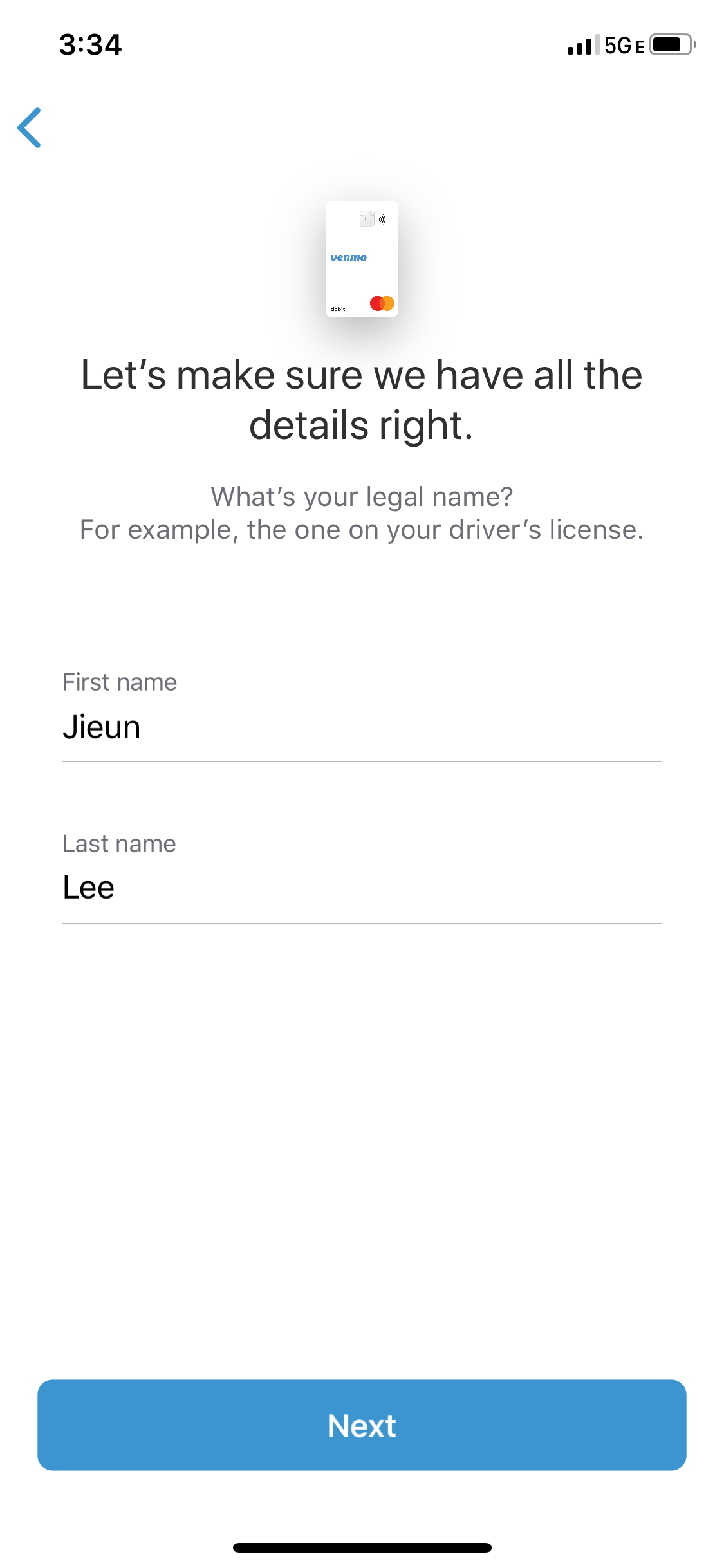The image depicts an iPhone screen showing a webpage or app interface that a user is interacting with. The top of the screen displays typical iPhone indicators, including the battery life, signal strength indicating 5G connectivity, and the current time, which is 3:34 PM. 

The main content of the screen appears to be a form, possibly part of a digital wallet or registration. The background of the form is white, and there is some branding present, including a logo in the lower right corner that looks like the MasterCard symbol, featuring its iconic red and yellow overlapping circles. Additionally, there is text that says "Welcome" alongside what seems to be an image of a credit card.

At the top of the form, there is a prompt in small gray print asking for the user's legal name, specifying that it should match the one on their driver's license. The user has started filling out the form: the first name entered is "Jieun," spelled as J-I-E-U-N, and the last name is "Lee," spelled as L-E-E.

Below the name fields, there is a prominent and unmistakable "Next" button designed to advance the process. This button is blue, spans the full width of the form, and features the word "Next" in bold white letters.